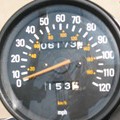This is a detailed zoomed-in image of a small, circular, black plastic speedometer with a glass cover. The background, visible around the corners of the speedometer, is light tan. The speedometer's face features a black background with white numerals ranging from 0 to 120 along its outer edge, incrementing by tens (0, 10, 20, 30, 40, 50, 60, 70, 80, 90, 100, 120). White dash marks, placed every five miles per hour, are located just inside these numbers. At the bottom, in white text, it reads "miles per hour".

Inside the circle, closer to the center, orange markings denote kilometers per hour, though they are somewhat difficult to read. The needle indicating the current speed is orange and pointed at zero. Above the needle's pivot point, there is an odometer displaying 06173, though the exact numbers are somewhat hard to discern. Below it, there is another smaller reading showing 153 in white text.